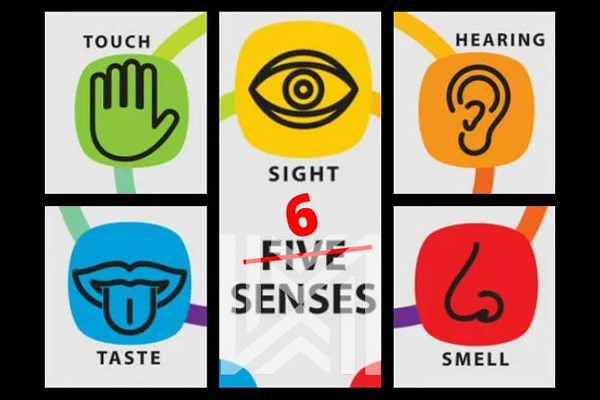This detailed image shows a poster board with a thick black outline dividing it into five distinct sections, each representing one of the five senses. The top-left section features a green hand icon with the word "Touch." Directly below it, the bottom-left section contains a blue box with a mouth and tongue icon labeled "Taste." The center section, which is notably larger and runs from top to bottom, includes an eye icon inside a yellow square at the top with the word "Sight" beneath it. Below this, the word "Five," which has been crossed out with a red line, appears, and above it is a bold red number "Six." The top-right section has an orange square with an ear icon labeled "Hearing," while the bottom-right section shows a red square with a nose icon labeled "Smell." The poster sits against a black background.